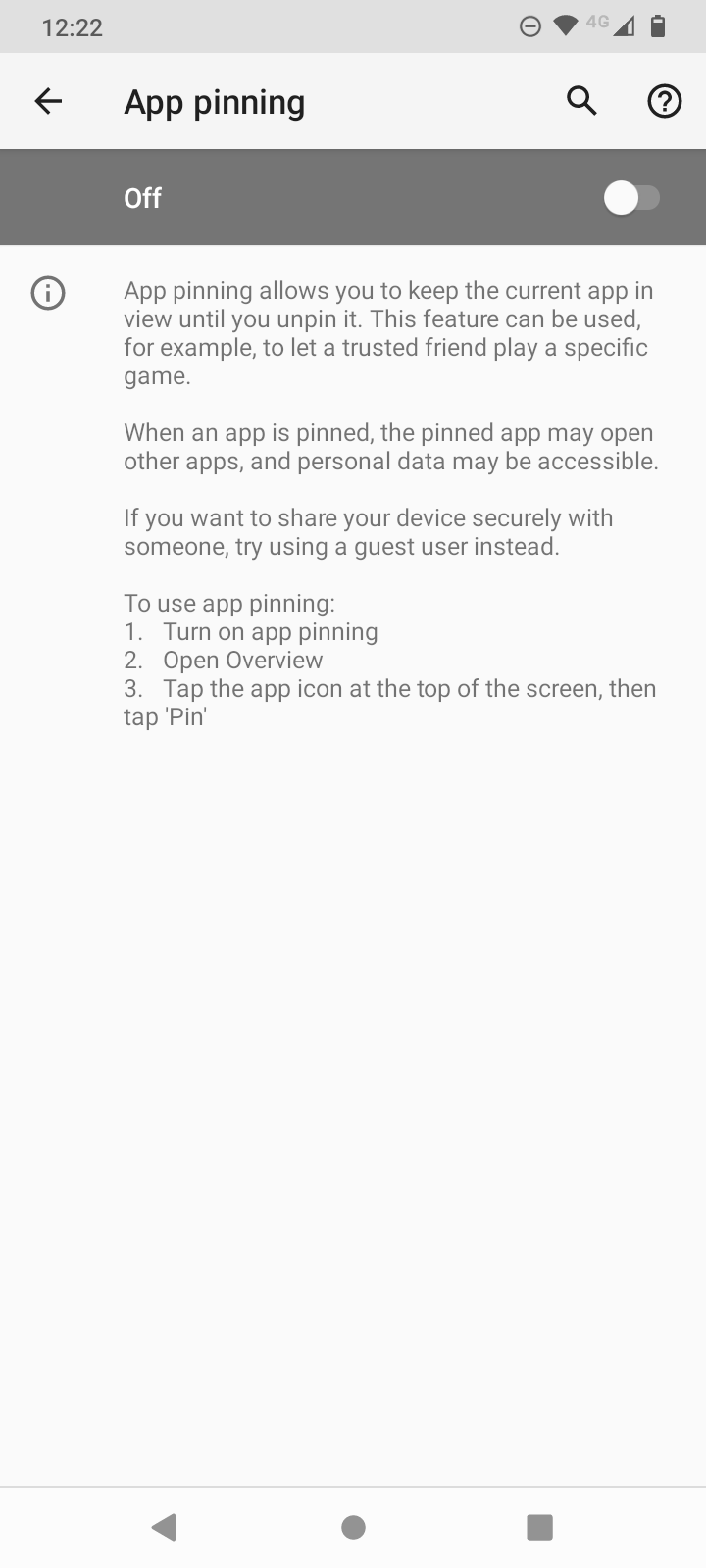In this image, the background is completely white, creating a clean and minimalistic look that highlights the phone's screen content. At the very top of the screen, there is an off-white header displaying several status icons. On the left, the time reads "12:22." On the right, there are multiple icons including a circle with a line through it, indicating a muted feature; a full Wi-Fi signal icon; the "4G" symbol denoting mobile network status; a cellular strength icon with halfway filled bars, and a battery icon showing approximately 75% charge.

Below this header, black text on the white background includes a back arrow pointing to the left, followed by the words "App Pinning." Next to this is a search icon and a question mark within a circle.

Underneath this text, there is a gray bar stretching across the width of the screen. Inside this bar, the word "Off" is displayed, indicating that the feature is currently disabled.

Below this gray bar, an informational section describes app pinning. An icon of an eye within a circle appears on the left, followed by the descriptive text: "App pinning allows you to keep the current app in view until you unpin it," with further detailed explanations continuing below.

At the very bottom of the screen, typical navigation icons are visible: a left-pointing arrow, a circle, and a square, completing the interface layout.